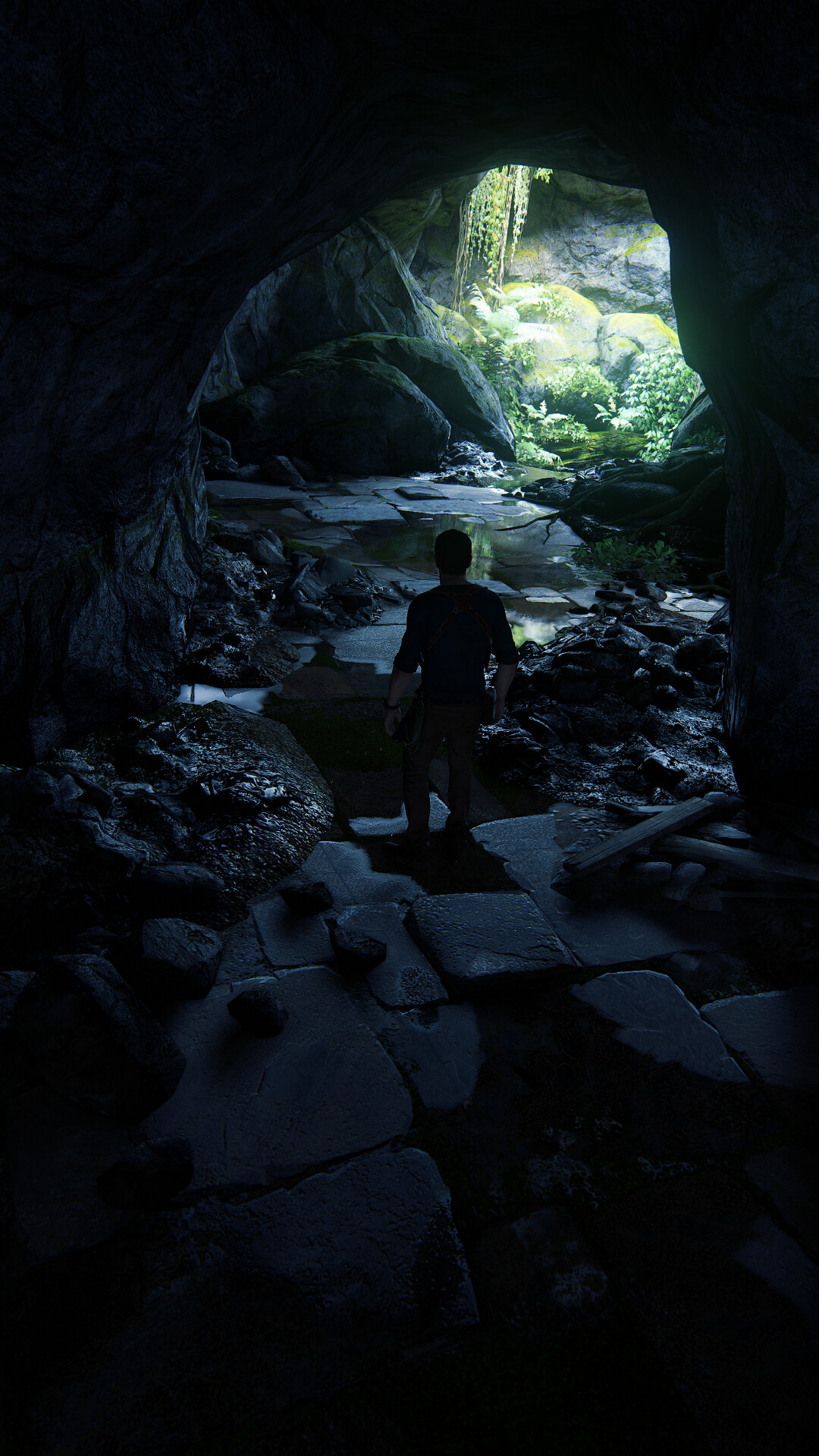In this stunning photograph, taken inside a breathtaking cave, a solitary man strides purposefully toward a radiant beam of light streaming down from an overhead opening. The cave's entrance or exit, visible in the distance, is bathed in natural sunlight, illuminating a lush green landscape that spills into the cave's depths. The foreground is enshrouded in darkness, revealing rugged, rocky formations that contrast sharply with the verdant, sun-drenched area at the cave's rear. Adding to the ethereal quality of the scene, shallow pools scattered across the cave floor mirror the rocks and greenery, enhancing the illusion of a CGI or AI-generated image. The brilliant reflections on the rocks and water create a surreal, almost otherworldly atmosphere.